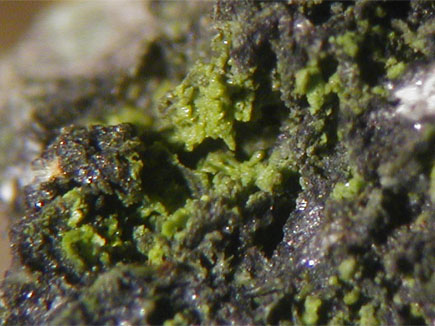This image captures an extreme close-up of a substantial amount of a light green and dark grayish-black sludge with a texture similar to chunky guacamole or mashed vegetables like broccoli or collard greens. The composition teeters on a build-up, sloping from the middle left to the top center area. The light green chunks suggest a hue close to avocado, contributing to 20% of the overall mass, while the predominant 80% is obscured in a dense, dark color reminiscent of liver. Scattered across this dark surface are what appear to be crystalline formations or glitter-like particles that catch the light. Notably, the right corner reveals some white fuzz, adding to the impression that this might be moldy guacamole. The photograph is so zoomed in that neither the type of container nor the immediate surroundings are visible, making the identification of the substance a mystery.